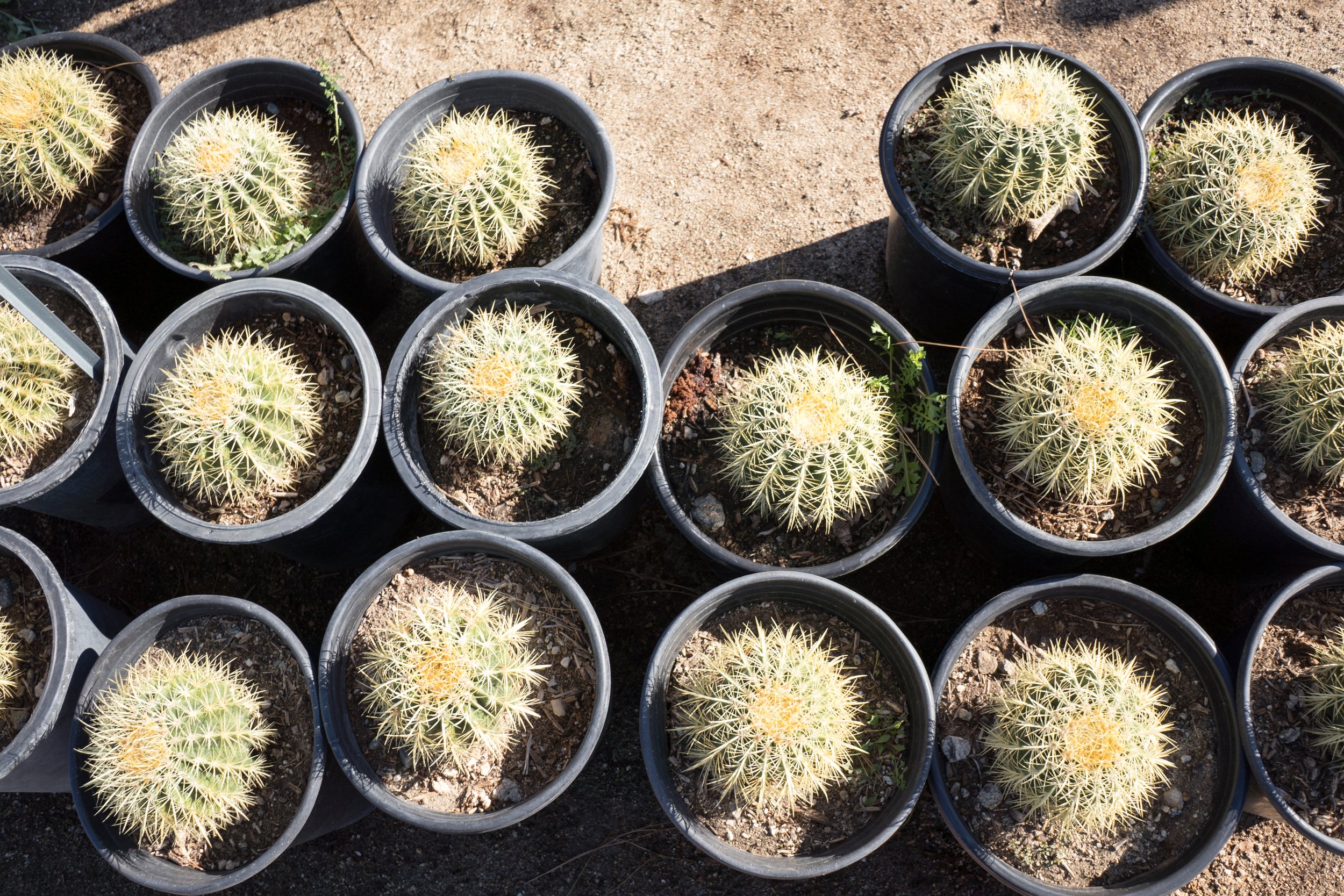This is a color photograph, taken outdoors in landscape orientation, capturing an overhead view of around 15 small cactus plants arranged in circular, charcoal or black plastic pots. The scene is set against a sandy, dirt background that hints at a sunny day, with visible shadows cast by the pots. The cactus plants are uniformly round and bulb-shaped, approximately the size of a small tangerine. Each dark green cactus features beige ridges running down its sides and is adorned with wispy, spiky beige needles, not appearing overly sharp. The top of each cactus showcases a distinctive yellow fuzzy area, adding a unique detail to their appearance. Several pots are partially cropped off at the edges of the photograph, reinforcing the naturalistic, representational style of the image.